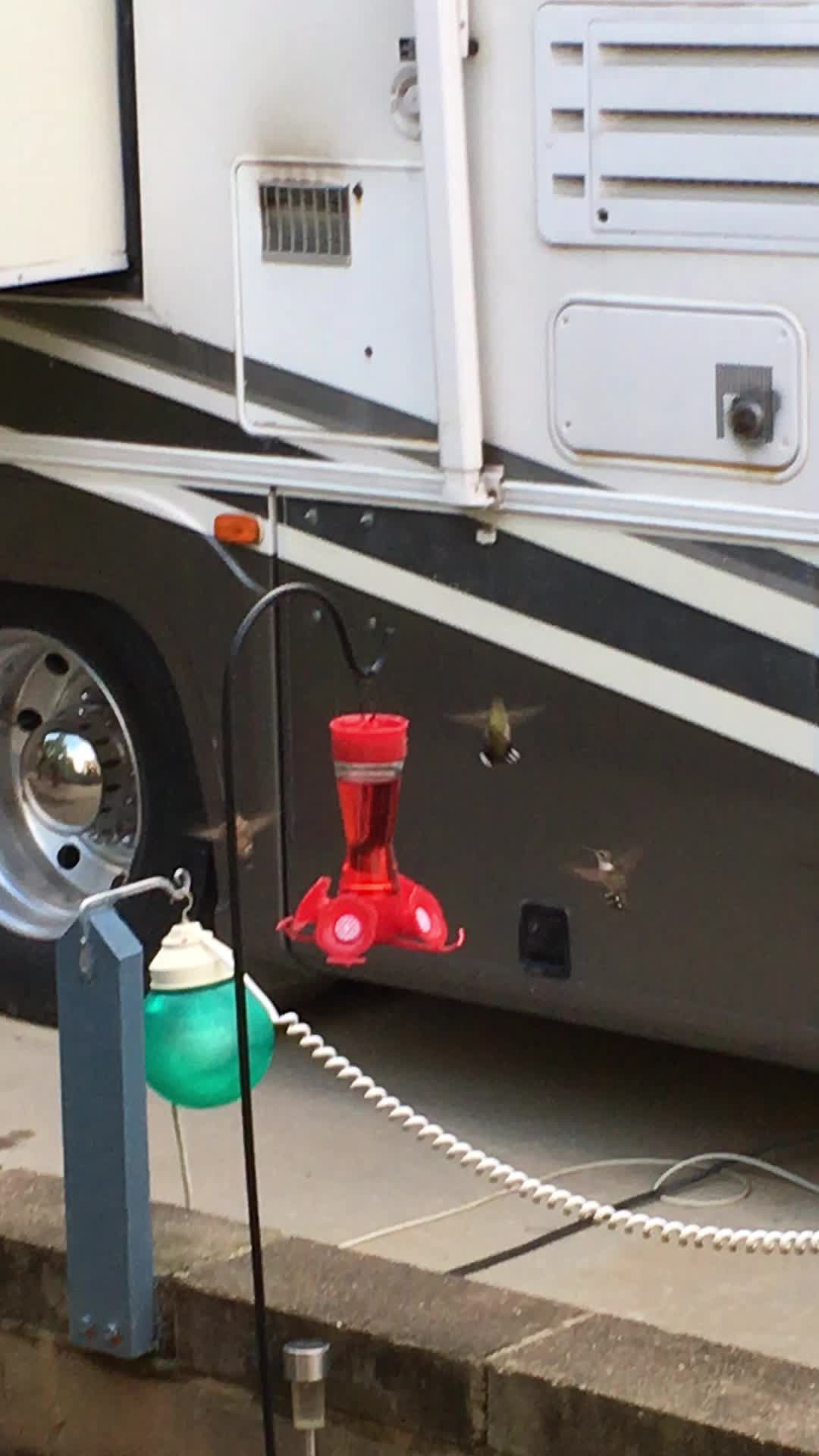The image portrays a vibrant outdoor scene centered around the side of an RV parked at a station. This RV features a color scheme of brown and white with distinctive stripes and a white top that includes compartments. In the foreground, a unique assortment of objects can be seen. Prominently, there's a green ball-shaped light bulb with a white tip, suspended from a blue support structure. A spiraled white cable extends from this light bulb and connects to the RV. Adjacent to the green light, an S-hook holds a red object, which appears to be a hanging bird feeder filled with water, possibly intended for hummingbirds. Three hummingbirds are visible, fluttering near the feeder, adding a dynamic and lively element to the image. The overall scene combines the earthy tones of the RV with the vivid colors of the various objects, set against the backdrop of an outdoor environment.